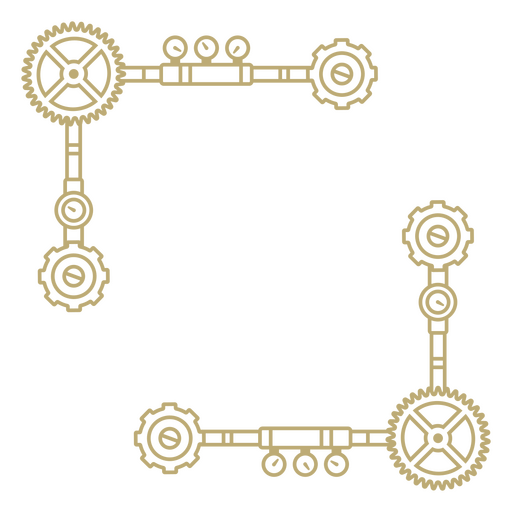The image features a white background adorned with a symmetrical arrangement of spiky, gold-colored cogwheels. Situated in the top left corner and mirrored in the bottom right corner, these cogwheels are interconnected with other gears, creating an intricate network that resembles sprockets and axles. Accompanying these cogwheels are numerous circular dials that resemble pressure gauges or barometers, complete with hands pointing in various directions. The overall design, composed of L-shaped structures made of pipes and gears, has a simple, schematic aesthetic, rendered in light tan and gold hues. This visually interesting graphic evokes the feel of a technical drawing or a stationary template.